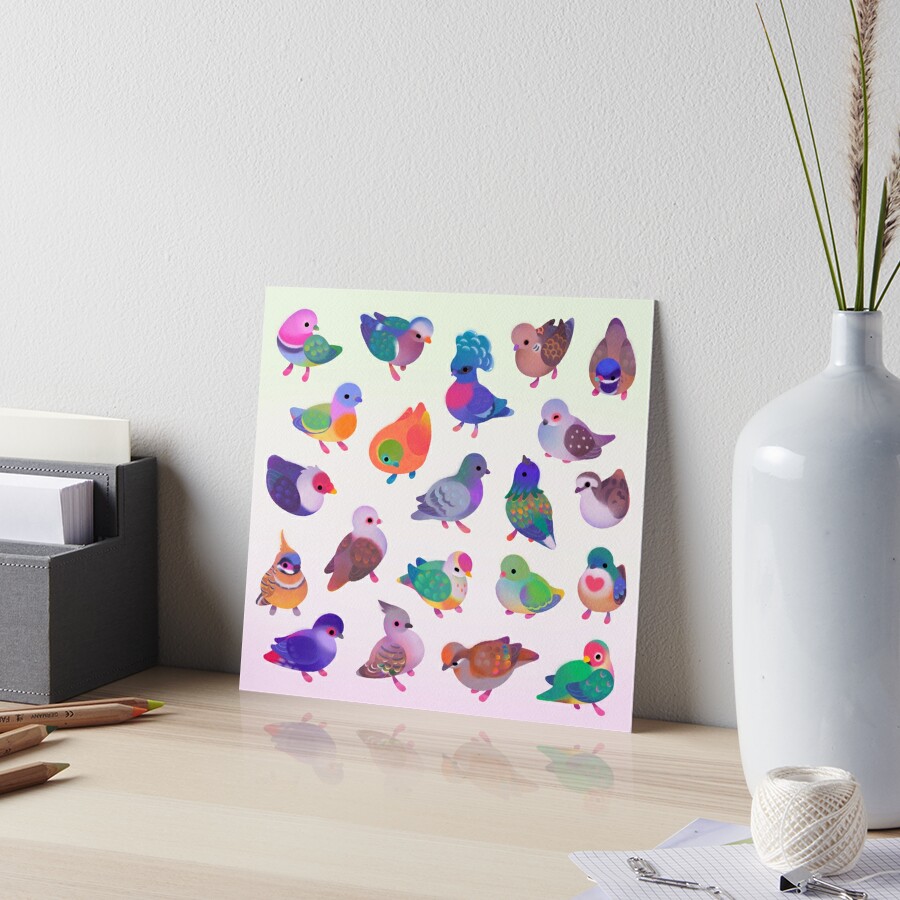This photograph likely taken in an art studio, showcases a light brown, shiny desk positioned at an angle in front of a plain white wall. At the center of the scene is a vibrant poster featuring approximately 20 hand-drawn birds, some whimsically decorated with hearts while others are rendered in realistic detail. The poster leans against the wall, casting a reflection on the glossy desk surface.

To the left of the poster, a gray fabric organizer containing envelopes or note cards is visible, with four colored pencils—potentially used to create the bird illustrations—strewn about nearby. On the right side, a sleek white vase holds about five fronds of green grass. In front of the vase lies a spool of thin twine, accompanied by paper clips and a binder clip. The desk arrangement, complemented by the vivid colors and delicate bird drawings, suggests an artist's workspace filled with creative potential and organized chaos.